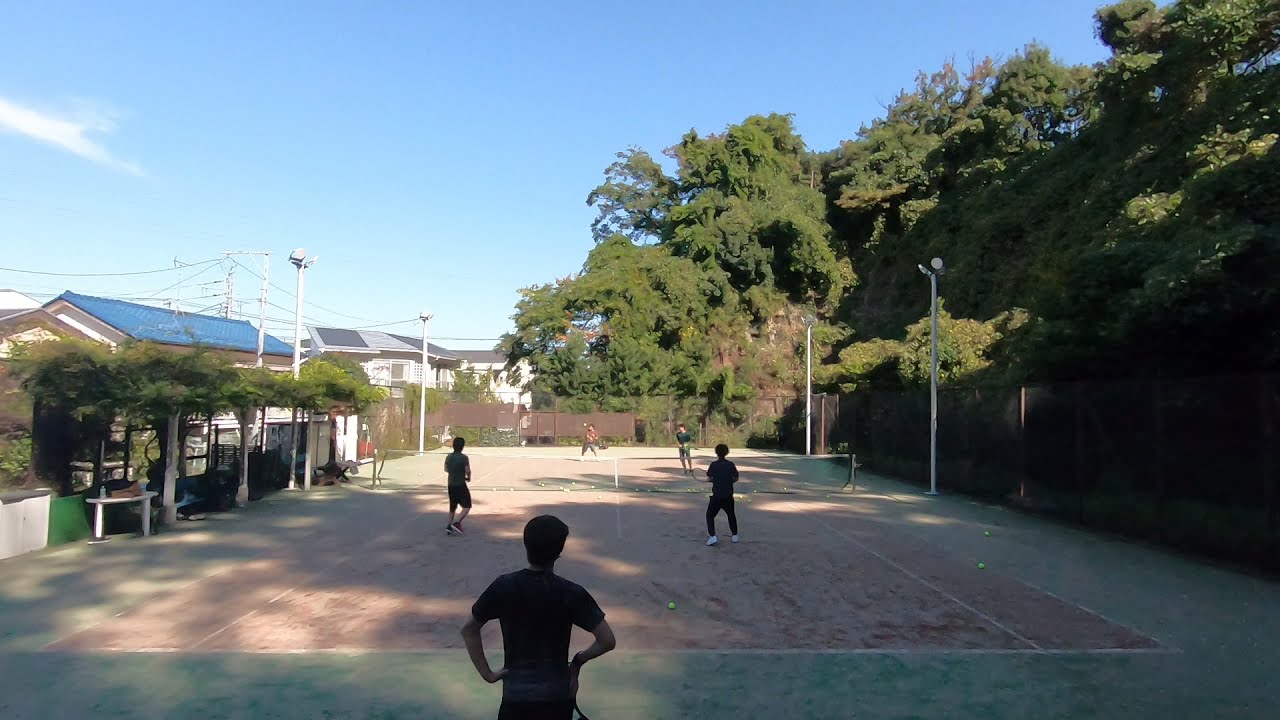The image depicts an outdoor tennis game in a suburban setting, viewed from a position behind the net. The court features a dusty reddish-brown surface and is surrounded by a green perimeter. Four players are engaged in the game, dressed casually in shorts and t-shirts, with numerous tennis balls scattered around the court. In the foreground, someone in a dark t-shirt stands watching the game. The right side of the court has a chain link fence backed by a steep, greenery-covered area, resembling a cliff. To the left, short trees provide shade near a small white wall and a white table. The background showcases buildings with white siding, some adorned with blue and gray roofs, and possibly solar panels. The blue sky above and abundant surrounding greenery indicate it is a bright, summer day.